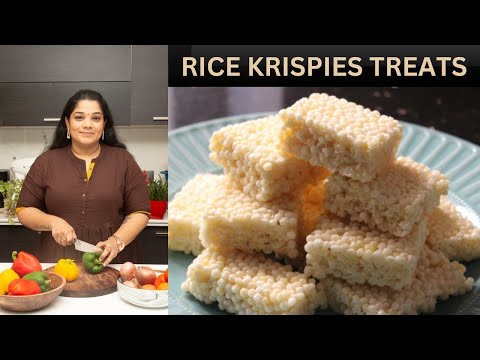In this vibrant kitchen scene, a woman with long brown hair, slightly heavyset, is the focal point on the left side of the image. She is dressed in a brown shirt with a yellow undershirt, accessorized with dangly earrings and a watch. The woman is caught mid-action, smiling warmly at the camera while cutting a green bell pepper on a round wooden cutting board. Surrounding her are various ingredients: yellow and green bell peppers on the board, a bowl filled with red, yellow, and green bell peppers, and another bowl possibly containing onions and additional red and yellow peppers. In the background, planters with fresh herbs add a touch of green to the kitchen’s lively atmosphere. On the right side of the image, in contrast to her culinary activity, a large blue plate prominently displays a stack of familiar Rice Krispie Treats. Above this plate, a banner reads “Rice Krispie Treats” in striking black and gold text. This juxtaposition highlights the dual focus of the image: the woman’s engagement in meal preparation with fresh vegetables and the tempting plate of sweet treats ready to be enjoyed.